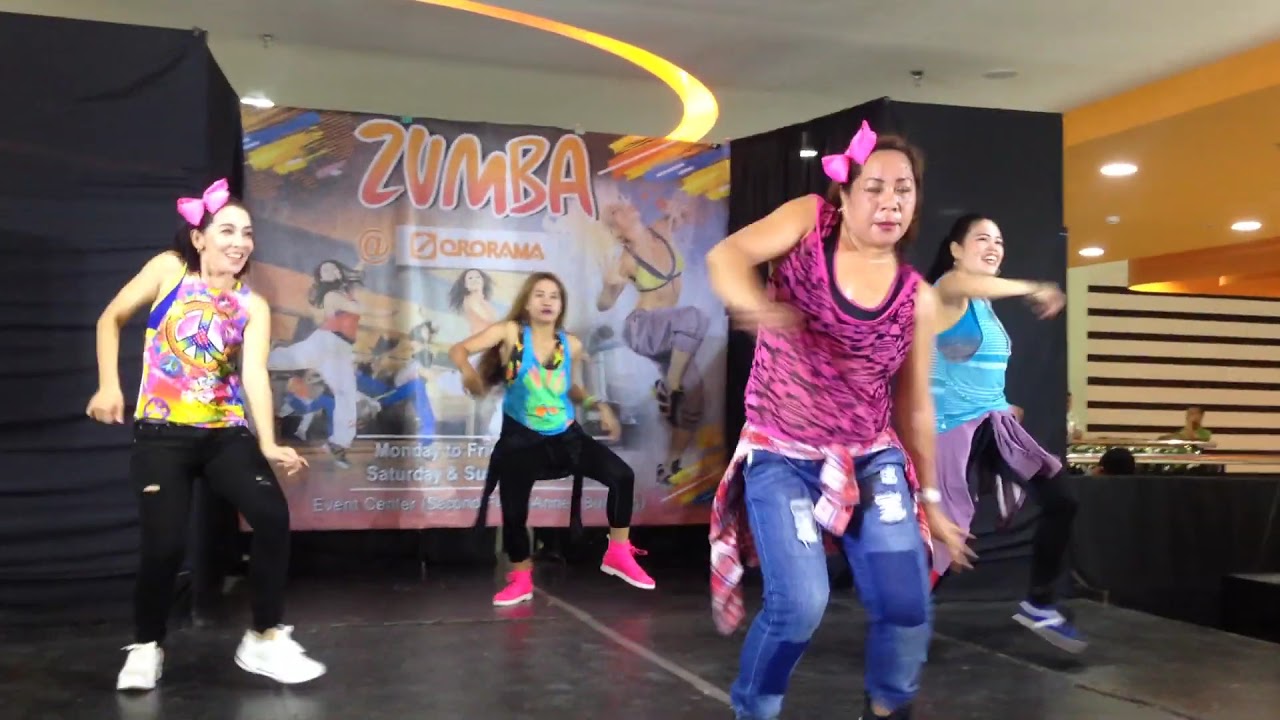A vibrant indoor scene captures a lively Zumba class consisting of pre-teen to adult Latina and indigenous women. The room features a large, prominent mural at the back, with the word "Zumba" emblazoned in bold orange letters at the top center, flanked by dancers in action. The women are dressed in tank tops and sports pants, each providing a splash of color and energy to the setting. In the foreground stands a teenage girl in a pink and black tank top with blue jeans, a pink bow in her hair, and a shirt tied around her waist. She is mid-dance, her right arm raised and left arm extended, exuding focus and determination.

Behind her, three women follow in what seems to be either a deliberate or accidental formation. To her left, a woman smiles, sporting a multicolored tank top, black pants, white sneakers, and a matching bow in her hair. Central in the back, another participant is energetically involved, wearing a blue top, black pants, and pink shoes. To her right, a woman appears mid-motion with a blue tank top, black pants, blue sneakers, and a purple sweater tied around her waist. Her raised hand and dynamic pose mirror the vigor of the class. 

The setting is a community center with a black tile floor, and the room is framed by two rectangular black blocks. The ceiling features built-in lights and an eye-catching yellow section that descends slightly with horizontal slats to the right. Additional text at the bottom of the mural suggests a community calendar, reinforcing the communal and inclusive atmosphere of the scene.